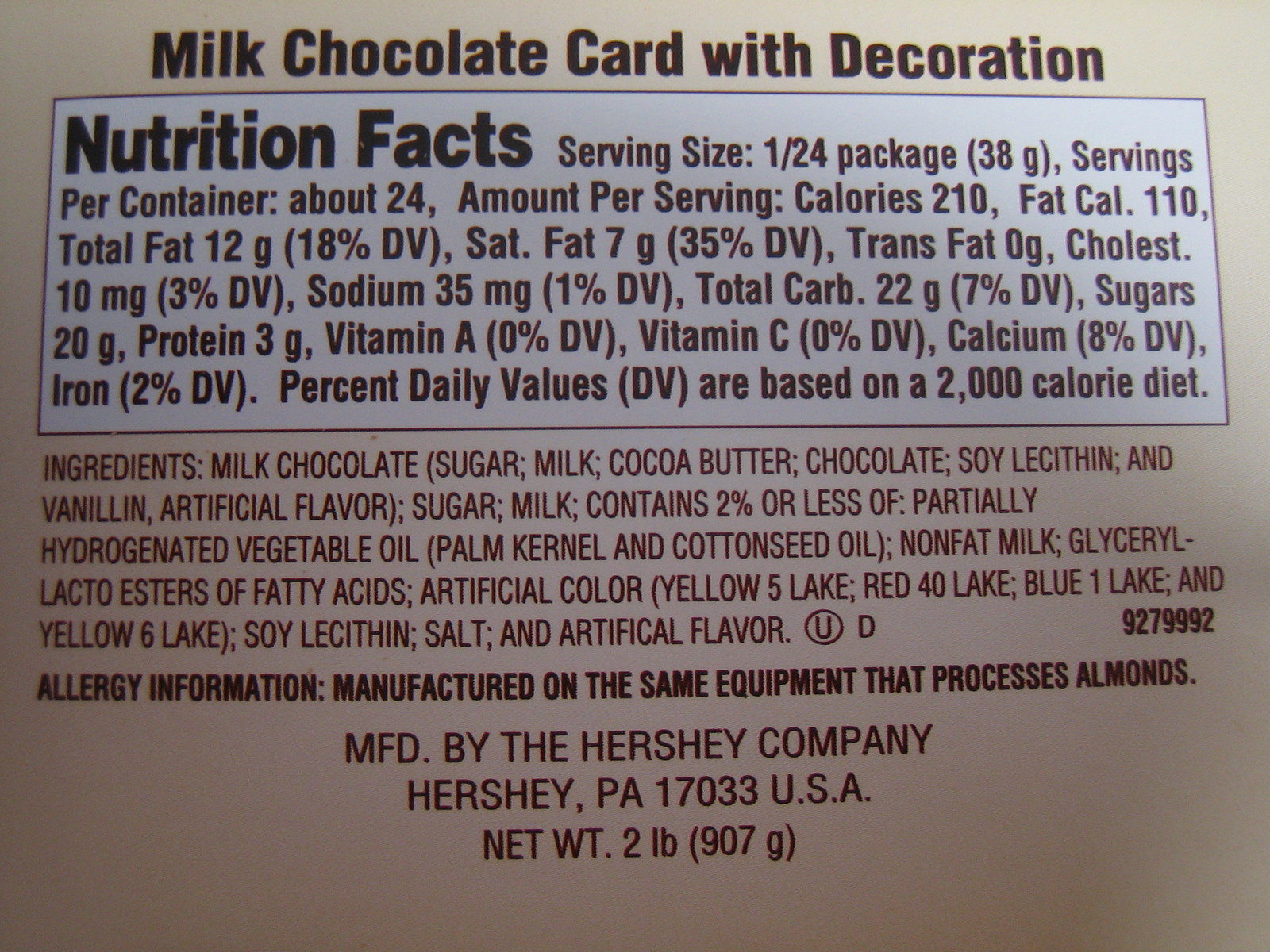This close-up image features a detailed nutrition label on a pale beige background. At the top, bold text reads "Milk Chocolate Cord with Decoration." Directly below, a white box highlights the Nutrition Facts, stating a serving size of 1/24th of the package (38 grams) with about 24 servings per container. Key nutritional details include 210 calories per serving. Beneath the nutrition facts, the ingredients are listed, starting with milk chocolate and followed by components in parentheses: sugar, milk, cocoa butter, chocolate, soy lecithin, and vanillin (artificial flavor). Additional information notes that the product is manufactured on equipment that processes almonds. The label also includes the manufacturing details: "MFD by the Hershey Company, Hershey, Pennsylvania 17033, USA." The net weight is noted as 2 pounds (907 grams).